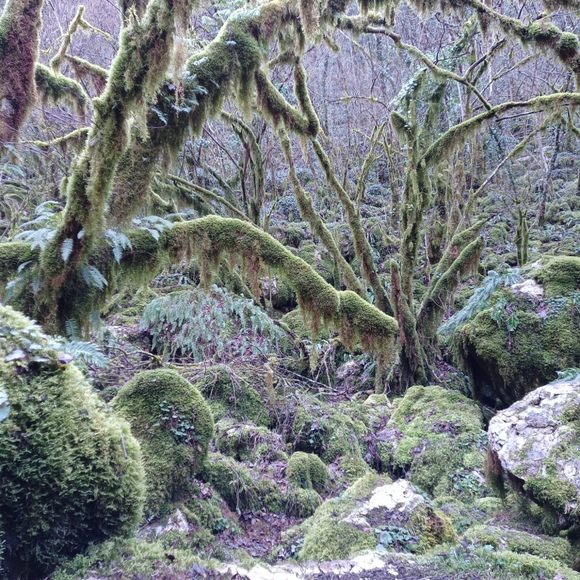The square-shaped image depicts an eerie, almost enchanted forest scene, characterized by a tapestry of thin, fuzzy, moss-covered tree limbs intertwined throughout the middle and upper areas. The backdrop, bathed in light purple hues complemented by patches of forest green, light blue, and white, creates a unique and somewhat abstract atmosphere. Moss and possibly lichen cloak the scene, giving the stones and trees a fuzzy, ethereal appearance. Two large, moss-covered rocks stand out on both the left and right sides, while further back, shades of brown and gray blend with the green and purple foliage. The ground is a mix of brown earth interspersed with green moss, enhancing the mystical and slightly eerie ambiance of this deep woodland setting.